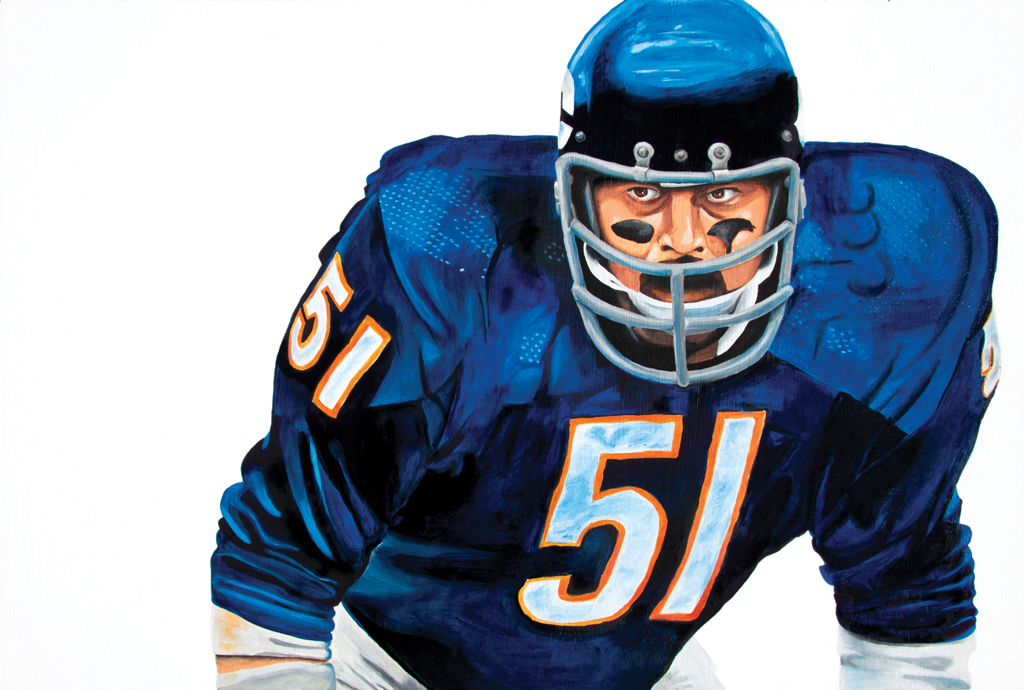This highly detailed and photorealistic artistic representation depicts a football player facing the camera while looking off to the left. He's adorned in a blue jersey with the number 51 prominently displayed in white with orange borders, both on his chest and sleeves. Underneath his blue shirt, he wears football padding, giving his shoulders a wide, thick appearance. His uniform includes white gloves and pants, though only his torso is clearly visible. The player's helmet is blue, accented with a gray metal face guard and a white chin strap, with a highlight that suggests a shiny surface. His skin tone is yellow, possibly indicating Hispanic or Pacific Islander heritage, and he has black grease marks under his eyes. The background of the image is white, further emphasizing the sharp, realistic details of his focused, serious expression.